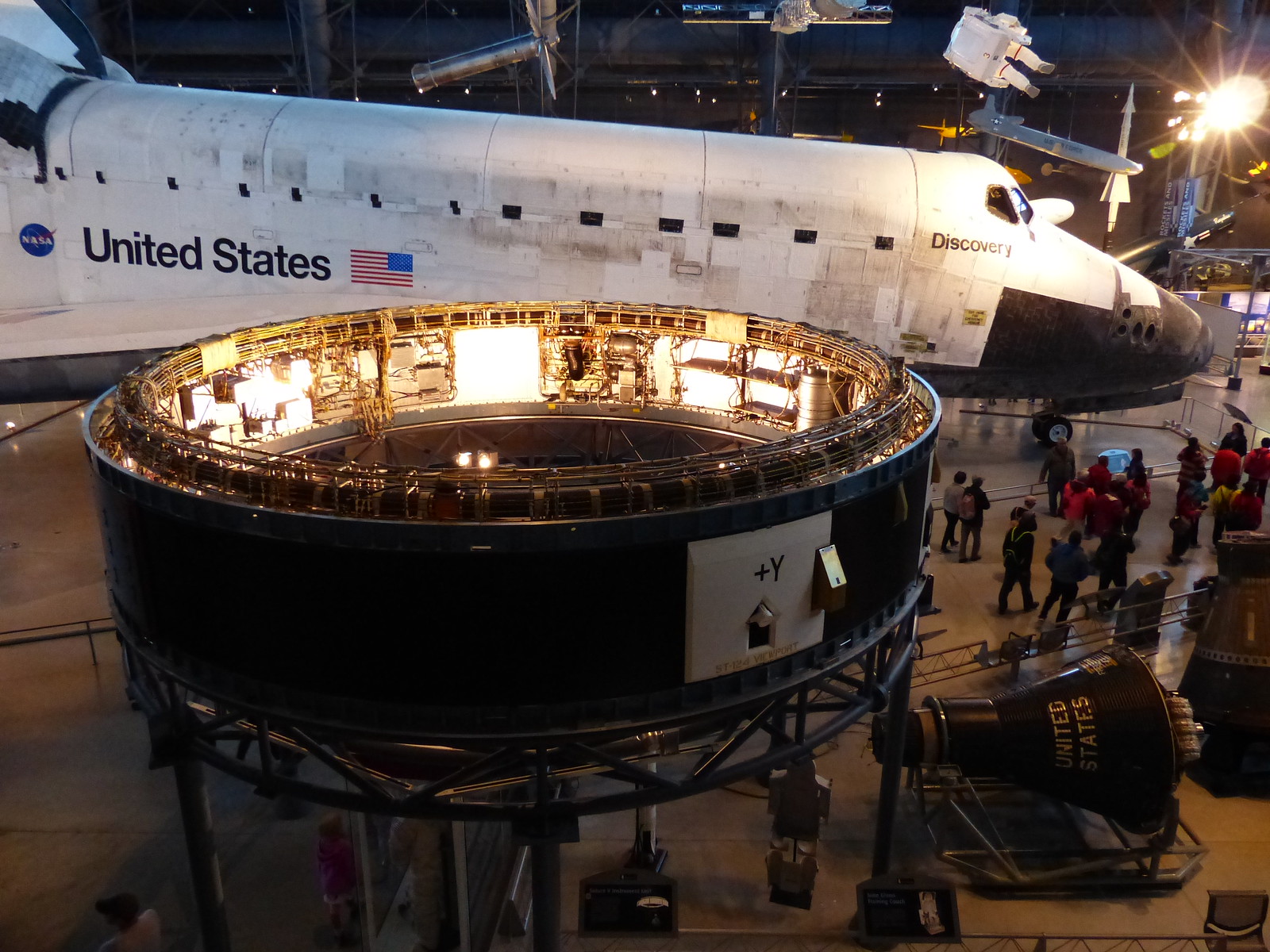This image showcases a white NASA space shuttle on display inside a warehouse or garage-like setting. The shuttle is prominently positioned in the background and takes up most of the frame, extending almost from one end of the image to the other. Marked with the text "United States" in black letters and a reversed American flag, the blue field of stars is oddly positioned at the top right. The NASA logo, a blue ball with "NASA" written in white, is visible to the left of the "United States" text. The cockpit area features the name "Discovery." In the foreground, there is a circular, dome-like component, possibly part of a launching pad, with illuminated lights and metal structures around it. A rectangular sign with "plus Y" and a stylized house-shaped cutout is also present. The space is bustling with many people—around 20—milling around and observing the shuttle. The ceiling features additional lights and technological equipment, enhancing the detailed and dynamic setting of the scene.